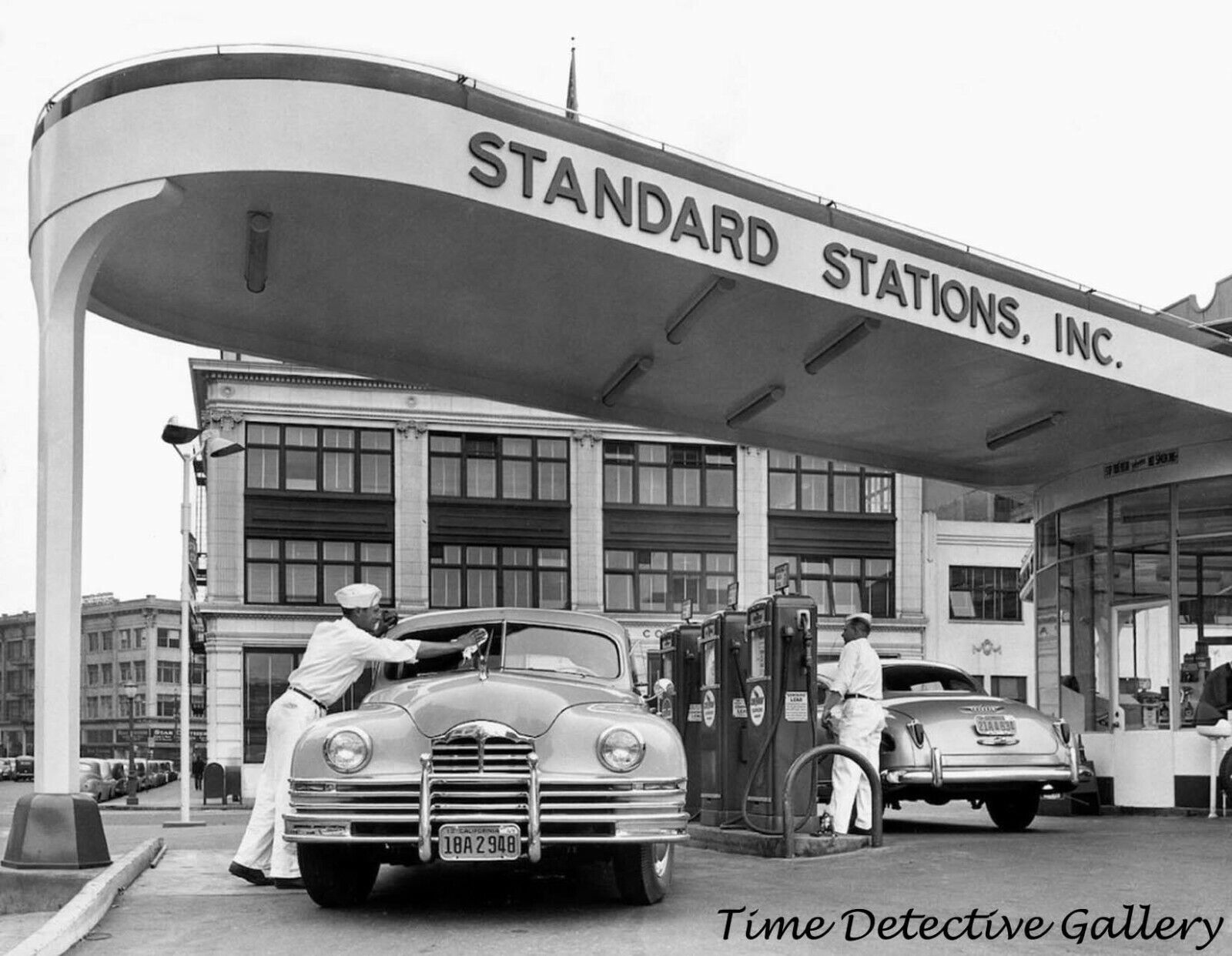The vintage black and white photograph captures a 1940s-era gas station named Standard Stations, Inc., prominently displayed in large black letters on the long, oval-shaped awning accented by black borders and neon tubing. Below the awning, two attendants in white uniforms resembling sailor outfits, complete with white caps and black shoes, are servicing two classic cars. The attendant on the left is polishing a windshield, while the one on the right is pumping gas. To the far right, a rounded, glass-lined store area is visible. In the backdrop, a small three-story concrete building with multiple glass windows can be seen. The photograph, part of the Time Detective Gallery collection, features its name inscribed in cursive black lettering at the bottom right of the image.